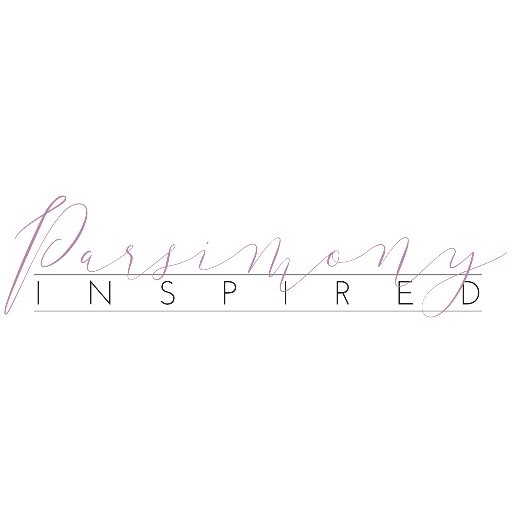The image depicts a minimalist white background featuring prominently the brand name "PARSINONY" written in a slightly purple cursive font, resembling delicate handwriting. Directly beneath "PARSINONY" is a distinct horizontal black line, accompanied by the uppercase word "INSPIRED," spelled out with large black letters spaced apart. Below "INSPIRED" lies another horizontal line, matching the purple hue of the cursive text above. The juxtaposition of the elegant script and bold, squared lettering gives an intriguing, yet unclear indication of the product being advertised, as no specific product (like perfume or handbags) is explicitly mentioned.